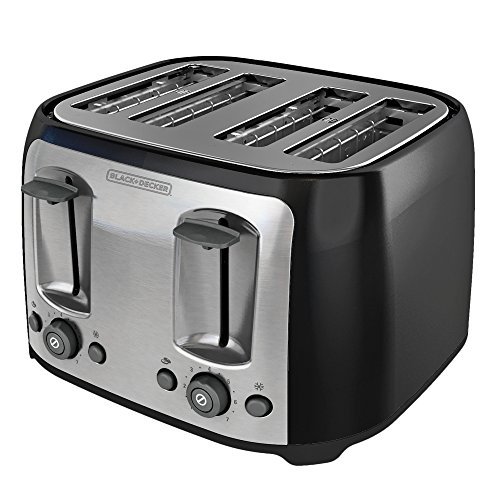This image depicts a Black & Decker four-slice toaster, showcasing a sleek and modern design. The toaster predominantly features a glossy black finish, complemented by chrome accents on the top and control panel. The control panel on the front displays the brand name "Black & Decker" prominently. 

Each side of the toaster is equipped with a manual lever for operating the slots, along with three buttons below each lever, providing a total of six control buttons. These buttons allow users to customize their toasting preferences. Below the levers, there are two dials, each surrounded by numbers ranging from one to seven, offering incremental heat settings for precise toasting.

The toaster's top section has four rectangular slots, each containing small grid-like wires that run horizontally and vertically to ensure even toasting. The overall shape of the toaster is rectangular, making it a stylish and functional addition to any kitchen.